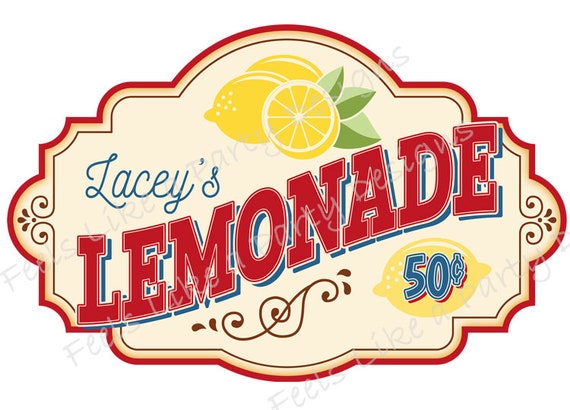The image is an illustrated advertisement for "Lacey's Lemonade" featuring prominently styled text and vibrant imagery. The word "Lacey's" is written in blue, cursive script, while "Lemonade" is splashed across the middle in a bold, diagonal fashion with dark red, capital letters. At the top center of the advertisement, three yellow lemons with green leaves are depicted, including one lemon cut in half to show its inside. Another yellow lemon appears at the bottom right corner, with the price "50 cents" written atop it in blue. The background is a pale pink, complemented by a red floral border. The entire image exudes a vintage feel with added blue outlines and faint watermarks that read "feels like a party" repeated at least three times across the advertisement. This detailed layout blends nostalgic charm with lively visuals, effectively capturing the essence of Lacey's Lemonade.